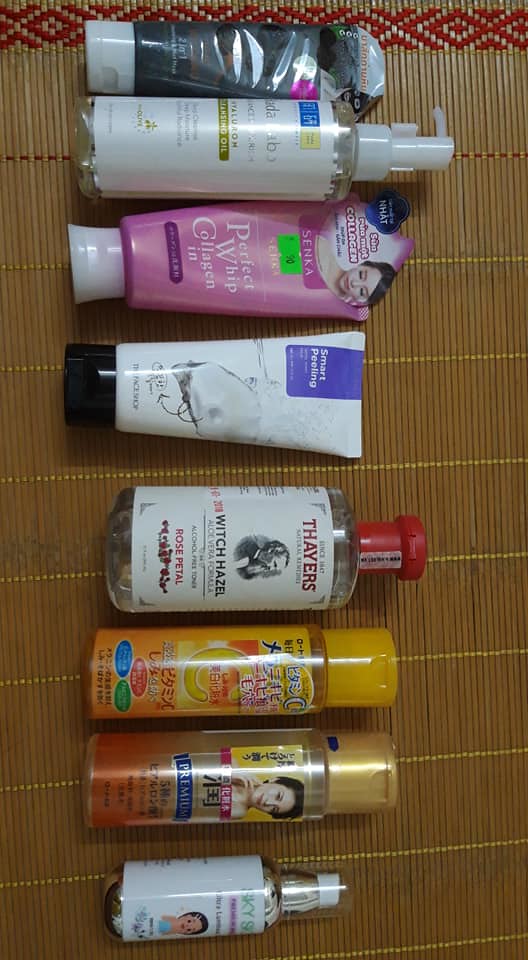Vertical image featuring an assortment of beauty products arranged in descending order. At the very top, there is a gray tube. Directly beneath it is a white pump bottle labeled with "something oil," followed by a pink tube that reads "collagen." Below the pink tube, there is a white tube with a black cap. Continuing down, there is a clear glass bottle with a red cap labeled "witch hazel." Beneath this are two orange bottles resembling shampoo bottles, each with an orange cap and Japanese lettering; one of these features an image of a woman. At the bottom, there is a white bottle with a silver label and a silver bottle with a white label. The collection includes various tubes, pumps, and shampoo bottles, showcasing a diverse range of beauty and skincare products.